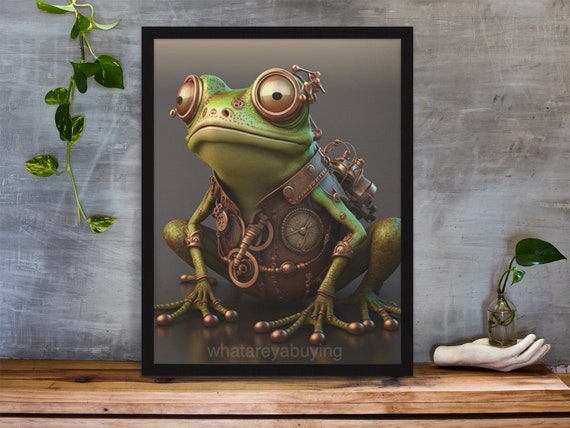The image is a detailed and visually compelling digital illustration framed in black, portraying a cyberpunk frog. The frog, predominantly green with brown spots, is adorned in a vest that extends to cover its lower body, detailed with numerous steampunk-inspired tubes, dials, and industrial machinery. The frog's body showcases several metallic enhancements, including metal fingertips and mechanical rings around its large eyes, which give it a distinct futuristic look. It carries a backpack equipped with tanks and intricate tubing.

In the digital artwork, at the bottom of the image, the phrase "what are you buying?" is photoshopped in a single line. The background of the framed picture is a textured gray wall, with some leaves of a plant trailing down from the top left corner. The entire framed illustration is placed on a small wooden table. To the bottom right of the framed picture, there is a ceramic sculpture of a hand holding a small glass jar, from which a plant is growing.